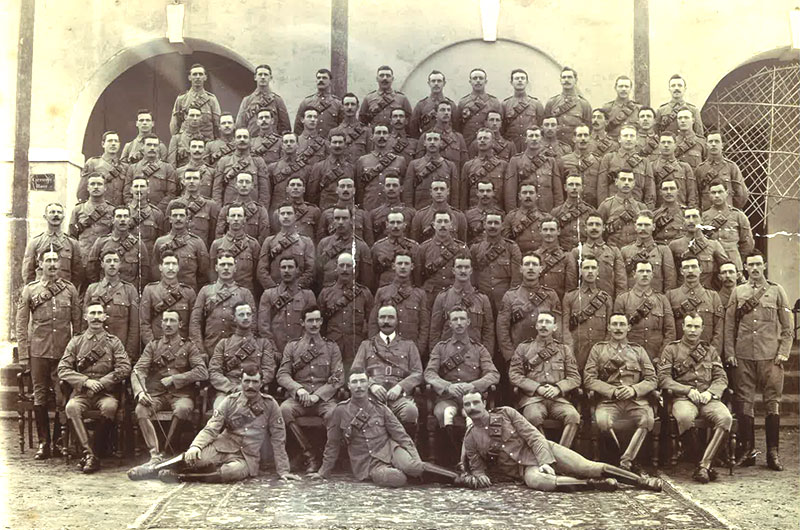This aged, black-and-white photograph, tinted with sepia, features a group of military men arranged in meticulously organized rows in front of a cement building with prominent archways. The photograph shows signs of wear, with frayed lines indicating it was once folded into four sections. The formation starts with three men sitting on a large 10 by 12 feet rug at the front; the two on the ends have their legs angled outward, while the man in the center directs his legs to the right. Behind them, the next row consists of men also seated on the bare ground surrounding the carpet. The subsequent rows rise progressively on risers or bleachers, creating an orderly, tiered structure that allows all individuals to be visible. Each man is dressed in a non-field military uniform, including a strap over the shoulder and tall boots reaching just below the knee. The backdrop and the precise arrangement evoke the atmosphere of a formal event or class photo within a military academy.